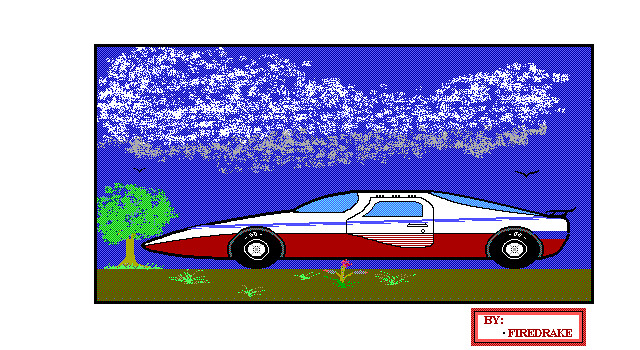This image is a detailed computer-enhanced drawing of a unique race car set against a vibrant backdrop. The car, appearing to be a hybrid design reminiscent of both a car and an airplane, sports a sleek and aerodynamic body with a sharply pointed hood. Its bold color scheme features striking red and white hues, complemented by a prominent blue stripe running down the middle. Only the right side of the car is visible, showcasing its four wheels and intricate design.

The scene is set against a bright blue sky, dotted with a few stylized birds and a smattering of fluffy, cloud-like shapes that resemble dots. In the foreground, a solitary tree stands prominently in front of the car, rooted in a patch of dirt with some sporadic grass growth. The entire composition exudes a digitally enhanced aesthetic, marked by vibrant colors and a slightly surreal, polished appearance.

Additionally, the bottom right corner of the image includes a mark or insignia, possibly indicative of the artist's signature or a branding element, featuring the term "5 fire drapes." This element further suggests the intricate digital enhancement of the original drawing, making the image a captivating blend of traditional artistry and modern technology.